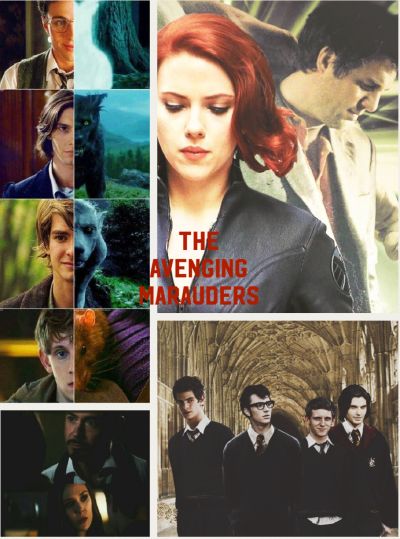This elaborate composite image resembles a movie or television show poster titled "The Avenging Marauders." Divided vertically, the right side features five distinct sections. At the top is an actress strikingly similar to Scarlett Johansson, with red hair and clad in a partially unzipped black top, set against a background featuring a suited man gazing downward. Below her, a quartet of teenage boys stands in a school hallway, attired in white shirts with ties and black cardigans, suggesting a uniform.

On the left side of the poster, five images present split-faced characters with their corresponding animal counterparts. From top to bottom, the first image shows a boy with a glowing white shadow. The second depicts a teenage boy next to a black wolf. The third portrays another boy alongside a gray wolf, while the fourth shows a younger boy with half his face as a mouse. The fifth image is dark and less clear, featuring a man and woman.

At the center of the image, bold red letters spell out "The Avenging Marauders," unifying the collage and hinting at a narrative intertwining human and animal identities.